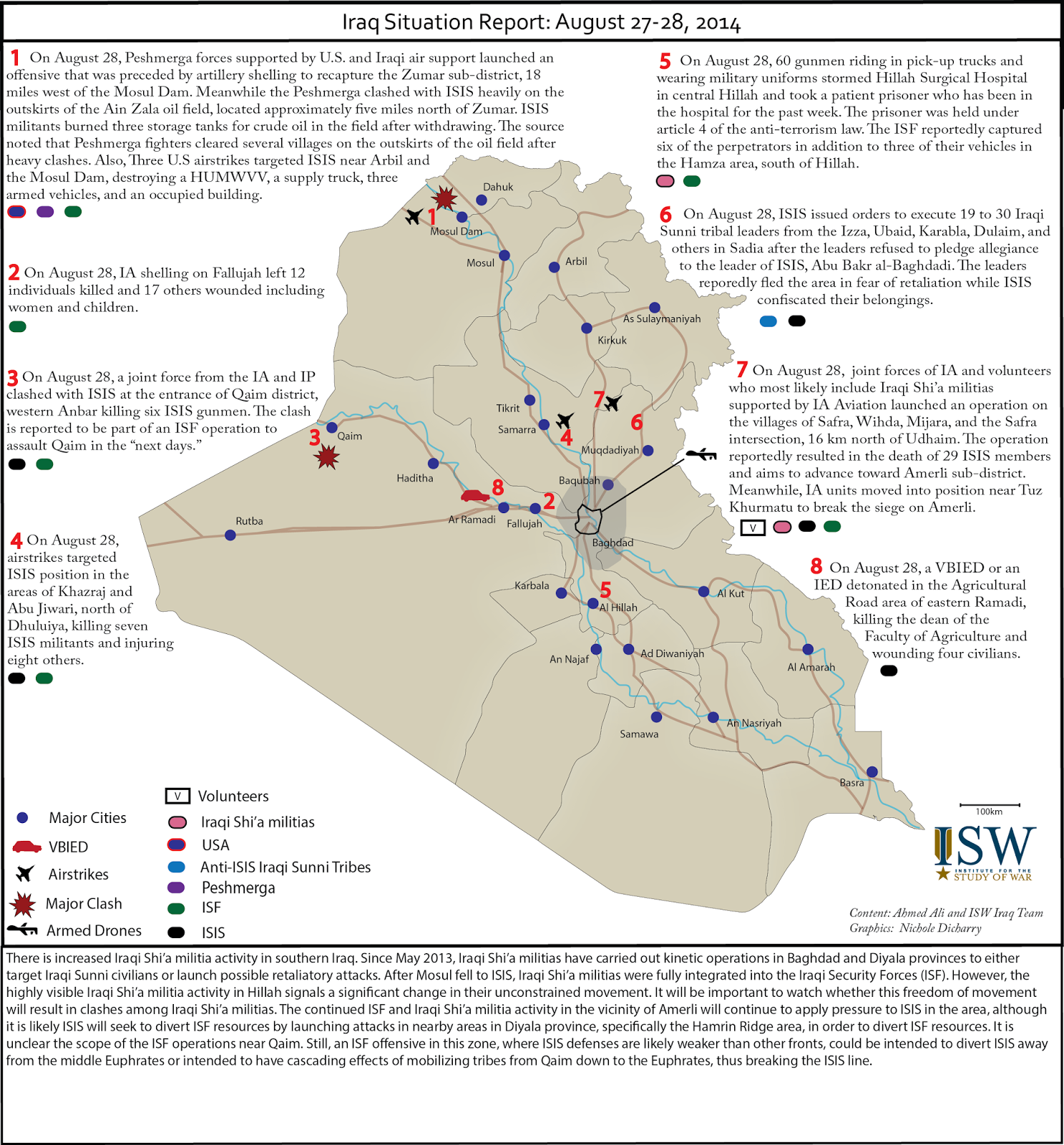The image depicts a detailed report titled "Iraq Situation Report" dated August 27, 2014. The report is structured into eight distinct points, each accompanied by a comprehensive paragraph outlining specific events and developments that occurred over a two-day period. At the bottom left corner, there is a legend featuring various symbols and terms, including major cities, Vehicle-Borne Improvised Explosive Devices (VBIED), airstrikes, major clashes, armed drones, volunteers, Iraqi Shia militias, USA, anti-ISIS efforts, Iraqi Sunni tribes, Peshmerga, Iraqi Security Forces (ISF), and ISIS. This legend aids in interpreting the report's detailed content regarding the complex military and political landscape during that timeframe.